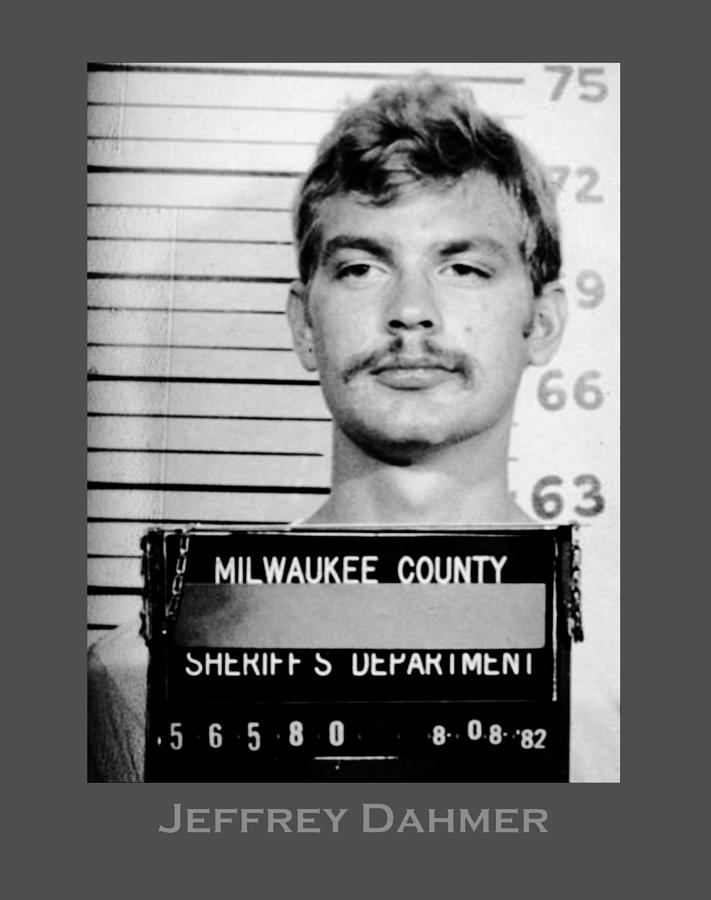This image is a black-and-white mugshot of Jeffrey Dahmer taken on August 8, 1982, as indicated by the date "80882" on a black sign with white lettering that Dahmer is holding. The sign also reads "Milwaukee County Sheriff's Department" followed by the identification number "56580." Dahmer, a white male with blondish hair and a thin mustache, stands against a height chart that measures from 63 to 75 inches, indicating he is approximately 6'1" tall. The mugshot captures only his head and neck, framed by a dark gray border with lighter gray lettering spelling out "Jeffrey Dahmer" at the bottom. Dahmer has a smug expression on his face and is looking slightly to the left.